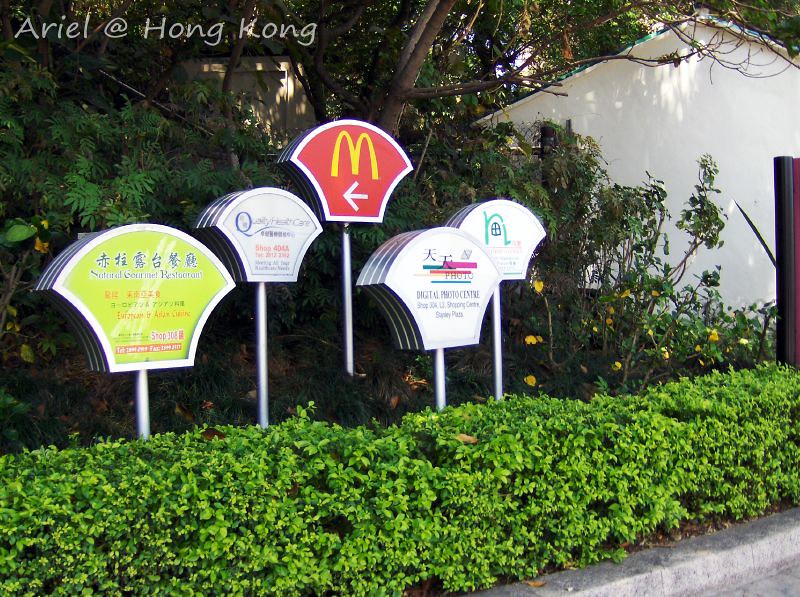This photograph, taken on a Hong Kong sidewalk, features a row of five distinctive signs against a backdrop of urban elements. At the top left, the image is labeled "Aerial at Hong Kong." Dominating the bottom of the scene is a short, green privet hedge that runs horizontally. In the lower right corner, a segment of a gray concrete curb is visible, hinting at a street or sidewalk setting. 

The five signs, each mounted on steel poles with frames, are planted in a landscaped area. The first sign on the left is green, advertising a restaurant, with blue lettering that includes both Asian characters and some English text. Next to it is a white sign promoting a company. The third sign stands out with its red background, emblazoned with the iconic golden arches of McDonald’s and an arrow pointing left. The fourth and fifth signs are also white, advertising different businesses. Each sign has a unique, badge-like shape: circular at the top and flattened at the bottom. 

To the right, the white stucco side of a building is partially visible, framed by a backdrop of lush trees. Additionally, yellow flowers can be seen surrounding the base of the signs, adding a splash of color to the green-dominated landscape.